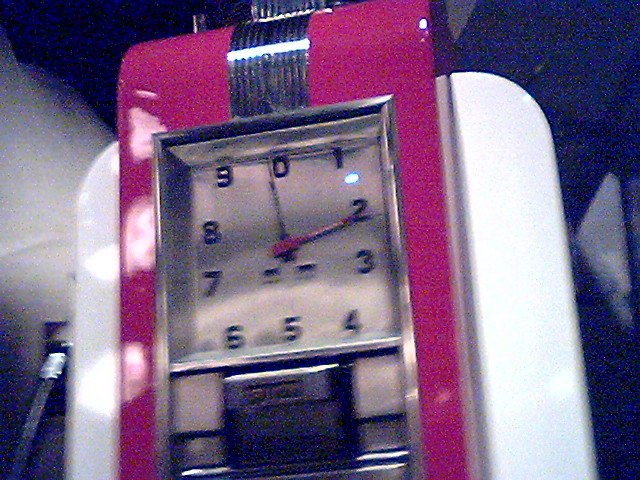The image depicts a unique, low-to-the-ground machine or case, featuring a large, central rectangular shape in a pinkish-red color. At the core of this shape, a clock or gauge with a silver stainless steel face is recessed, characterized by bold numbers ranging from 0 to 9. The clock has two hands: a red hand pointing to 2 and a black hand, with a prominent blue light situated between the numbers 1 and 2. Below this clock is a small hatch or handle. The red shape is enveloped by rounded white extensions on the sides and underneath, giving the appearance of being mounted on a white platform. A black hose is visible on the left side, suggesting the possibility of the object being a type of pump or vending machine, amidst a backdrop that transitions from black to gray.